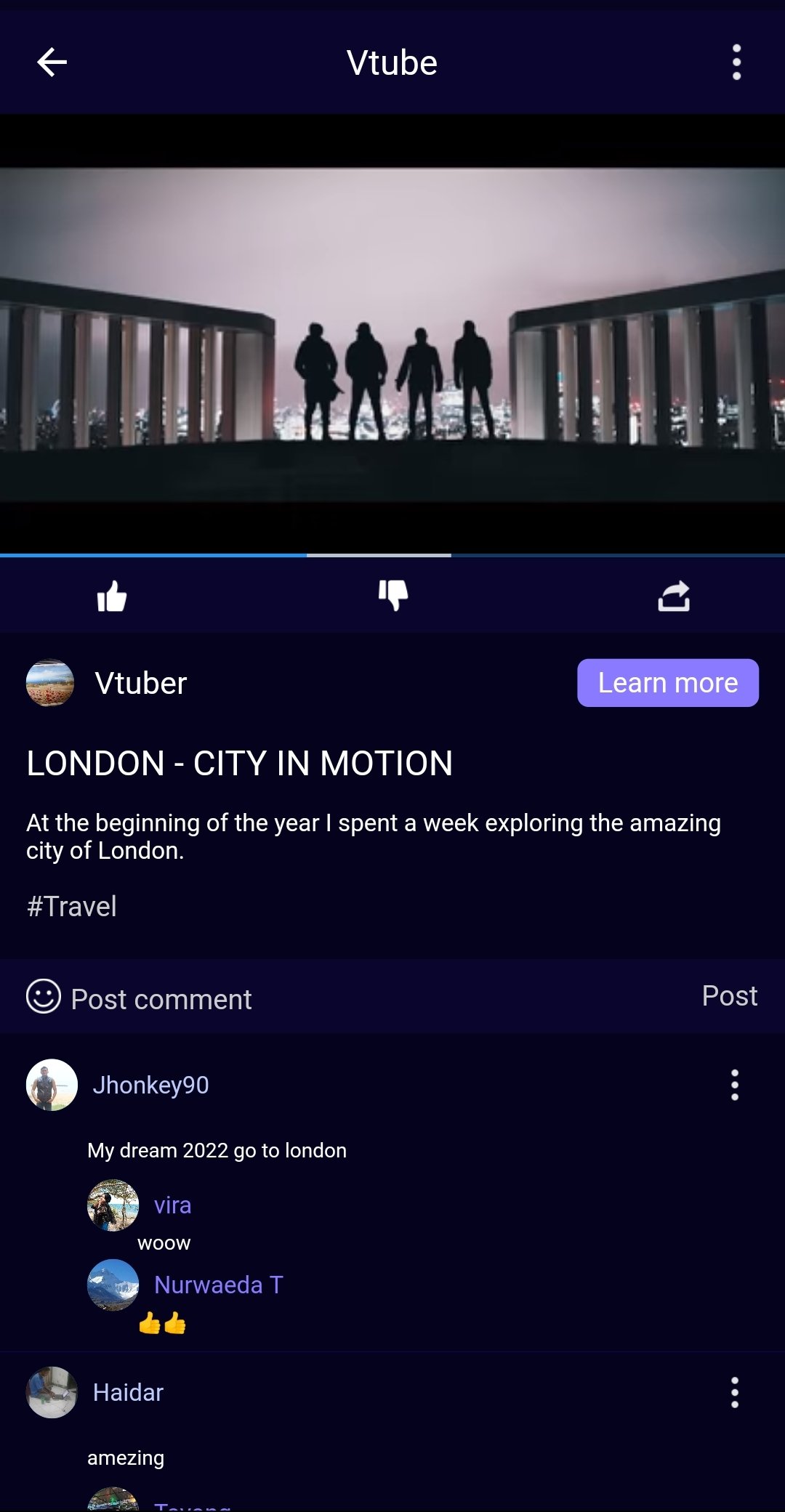This image is a screenshot from a phone, featuring a dark blue background. At the top left corner, there is a white arrow pointing to the left. Centrally positioned at the top is "V-tube," and on the right, there are three white dots aligned vertically. The image also includes a black border framing the main content.

The central part of the screenshot shows a gray sky with concrete columns extending about one-third inward from both the left and right sides. In the center, four silhouetted men are standing. A thin blue line runs horizontally just below the midpoint, with alternating sections of gray and blue beneath it.

Below the main image content, there are icons including a white thumbs-up, a white thumbs-down, and a share icon. Further down, a profile picture resembling a sky and brown earth is visible, next to the name "V-tube." To the right of this, a purple tab with the text "Learn More" in white is displayed.

Under this section, the text "London-City in motion" appears in white. Beneath this headline, additional text reads: "At the beginning of the year, I spent a week exploring the amazing City of London." Following this is a hashtag "#travel" in a lighter blue color.

Further down, the comment section begins with a lighter blue command line reading "Post comment," accompanied by a smiley face emoticon to the left and a "Post" option on the right. Various profile pictures with associated comments follow:

- One comment says: "my dream 2022 to go to London."
- Another, underneath the profile pic labeled "Fira," reads: "W-O-O-W."
- Another comment, under the profile pic labeled "NURWAEDA T," shows two thumbs-up icons.
- The next comment, though hard to make out due to the small size of the profile pictures, reads "amazing," accompanied by a white, vertically aligned three-dot icon on the right side.

This detailed screenshot provides a window into an interaction on the platform, showcasing user engagement and reactions to posted content.